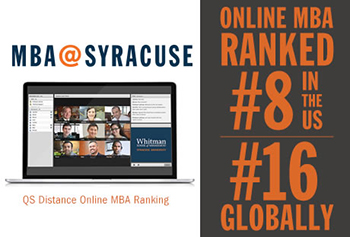This image is a detailed screenshot of a website or digital advertisement promoting the MBA program at Syracuse University. The top of the image prominently features the heading "MBA at Syracuse," setting the context. Below this heading, there is a visual element – an open laptop, which displays a page with nine individuals, though the specifics of this page are not clearly legible. To the upper right of the laptop screen, there is some text which is indistinct. Below the laptop image, a blue box with "Whitman" is visible, presumably referring to the Martin J. Whitman School of Management. Beneath this blue box, the text reads "QS Distance Online MBA Ranking." Occupying the right side of the screenshot, there is a brown box with bold orange letters stating, "Online MBA ranked number 8 in the US." A horizontal line under this information is followed by additional text reading "Number 16 globally," emphasizing the program's high ranking. Overall, this image appears to serve as an advertisement for Syracuse University's Online MBA program, highlighting its prestigious rankings both nationally and globally. It could feasibly be part of a web page or a digital poster.